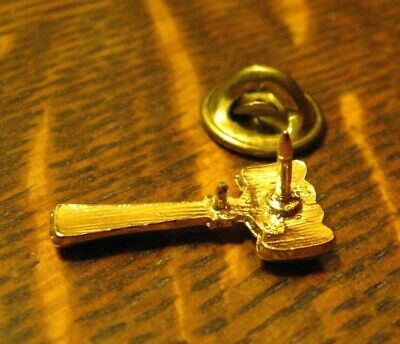The photograph, taken indoors, showcases a close-up view of a lapel pin designed to resemble a gavel. The image, with a warm yellow hue, highlights the golden lapel pin placed prominently at the center on a brown, wood-grain surface. The pin is positioned horizontally with the gavel’s handle on the left and the hammerhead on the right, while the central sharp needle of the pin points upward. A circular button-like pinback is spotted above the gavel head. The wood surface features dark brown and black grains, adding a contrasting backdrop to the intricate details of the golden pin. The overall composition and texture of the photograph elegantly capture the pin’s ornamental nature.